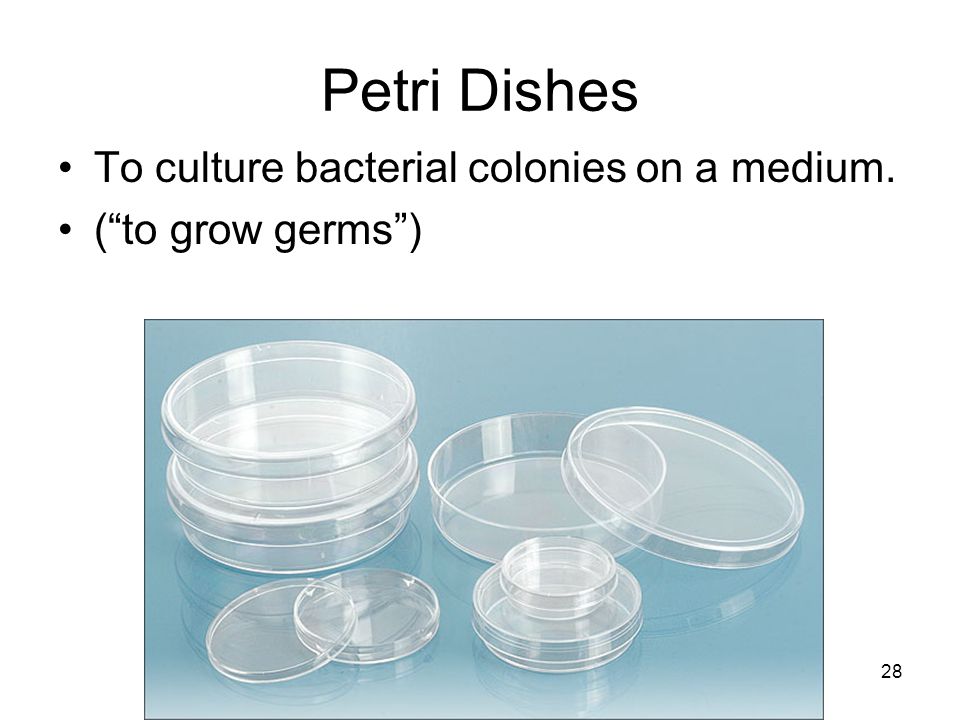The image depicts an assortment of Petri dishes with varying types of lids arranged on a blue background, likely used to culture bacterial colonies on a medium. At the top of the image, there is text that reads "Petri dishes," followed by a description that explains their purpose for growing bacterial colonies, with a simpler explanation in parentheses for clarity. The composition of the image suggests it could be a page from a book or a slide from an educational presentation, as indicated by the presence of a page number in the bottom right corner. The Petri dishes are located at the bottom center of the image. The collection includes three larger Petri dishes with standard lids, one smaller Petri dish, and one Petri dish featuring a more elaborate lid with a handle. The color palette of the image includes shades of black, white, blue, and gray.